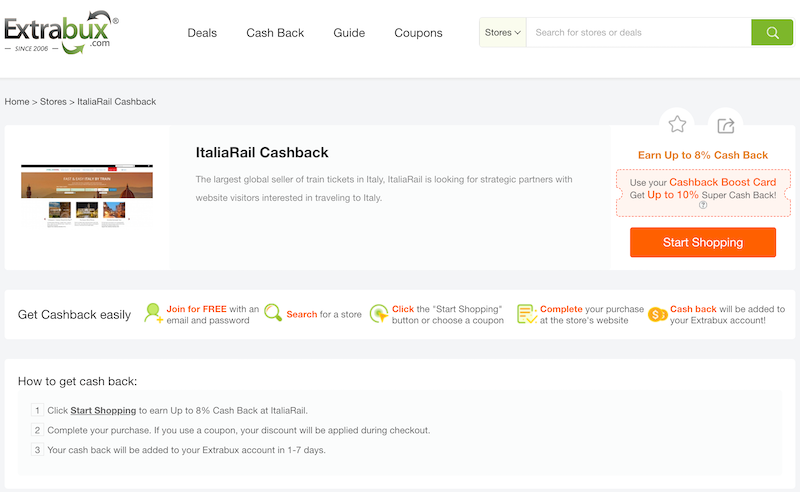Here is a descriptive and detailed caption based on the provided voice description:

---

**Screenshot Description of ExtraBox.com Homepage Featuring Italiarail Cashback Offer**

The screenshot captures the homepage of the website ExtraBox.com. At the top left corner, the logo "ExtraBox" is prominently displayed, with "Extra" in black and "Box" in green. The logo includes two arrows, one at the bottom and another at the top, which encircle the text towards the end. Below the 'X' in "Box.com", a slogan reads, "Are you seeing gray since 2006".

The top navigation menu includes four primary options: Deals, Cashback, Guide, and Coupons. Directly beneath this menu, the page focuses on the Italiarail Cashback offer.

An upper banner section features an image on the left, highlighting the Italiarail Cashback offer. The title "Italiarail Cashback" is written in bold font. Below this title, a brief description states, "the target seller of train tickets in Italy," and mentions Italiarail's search for strategic partners who have website visitors interested in traveling to Italy. To the right of this description, a prominent "Start Shopping" button encourages users to begin their shopping experience.

---

This caption provides a clear and concise description, detailing the layout, content, and features visible in the screenshot.